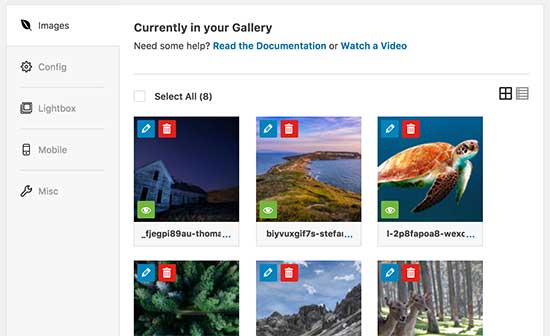This screenshot features a gallery interface with a navigation panel on the left-hand side displaying several categories: "Images" (selected), "Configuration" accompanied by a settings icon, "Lightbox" next to a gray box symbol, "Mobile" with a phone icon, and "Miscellaneous" represented by a wrench icon. Below this, text reads: "Currently in your gallery. Need some help? Read the documentation or watch a video."

The gallery itself contains six images:

1. An eerie nighttime photograph of an old, dilapidated farmhouse with shattered windows, indicating it has been abandoned for a long time.
2. A striking dusk shot of a peninsula extending far into an ocean, functioning as a breakwater. The sky is painted in hues of purplish-red and blue.
3. A vivid image of a sea turtle with a brown shell. The underneath of its shell and neck is aqua, with its flippers adorned in brown and dotted with black spots.
4. A bird's-eye view of lavender plants that appear on the verge of blooming, yet they haven't fully budded out.
5. A dramatic photograph of a rugged mountain range under an ominous, heavily clouded sky, suggesting imminent rain.
6. A serene forest scene featuring two deer – a doe and a young male with budding antlers.